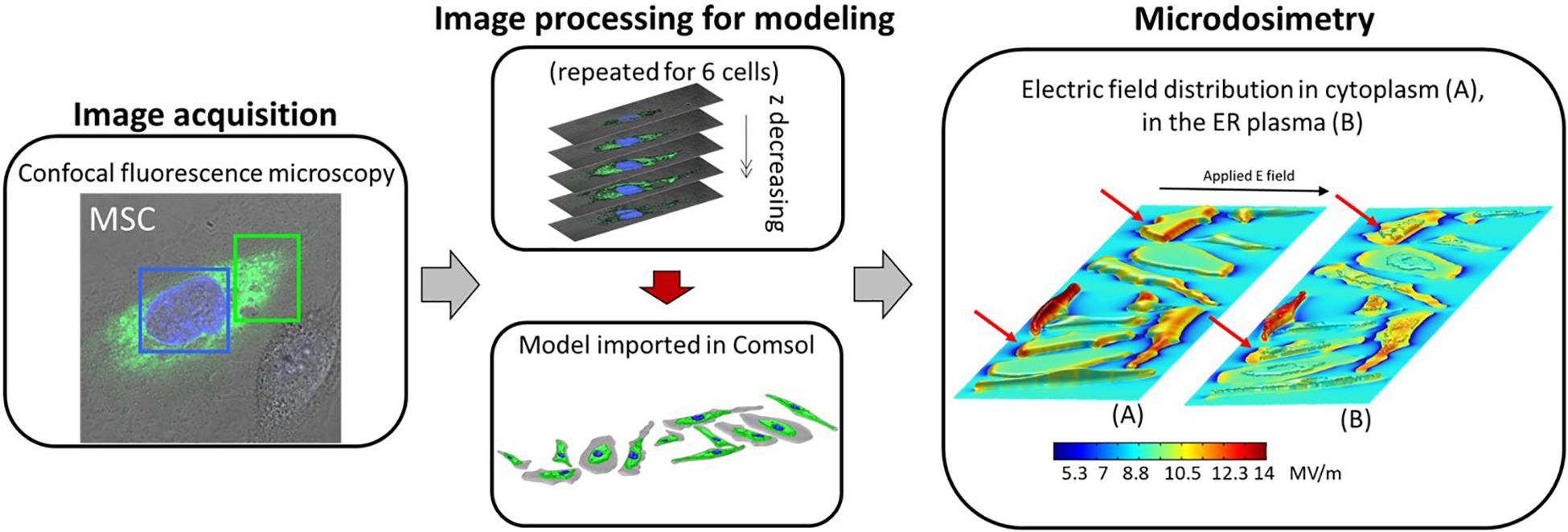The illustration is a detailed diagram with a white background, comprising four distinct sections each framed by rounded rectangles and connected by thick gray arrows. The diagram starts on the left with a section titled "Image Acquisition," featuring a gray square that contains two small boxes outlined in blue and bright green, labeled "MSC" in white uppercase letters. Above this, the text "Confocal Fluorescence Microscopy" is displayed.

An arrow leads to the next area in the middle, which contains two stacked rectangles under the heading "Image Processing for Modeling." Each rectangle has a white background with various images, displaying different colors and stacked rectangular forms in blue and green hues.

Another thick gray arrow points to the final section on the right, labeled "Micro Dosimetry." This larger rectangle includes multicolored geometric shapes, a color bar, and labels indicating "Electric Field Distribution in Cytoplasm" and "ER Plasma." The colors within this section are vivid, featuring blue, yellow, and red shades that illustrate specific data points.

Overall, the diagram showcases a sequential flow of image acquisition, processing, and modeling, leading to detailed micro dosimetry analysis.